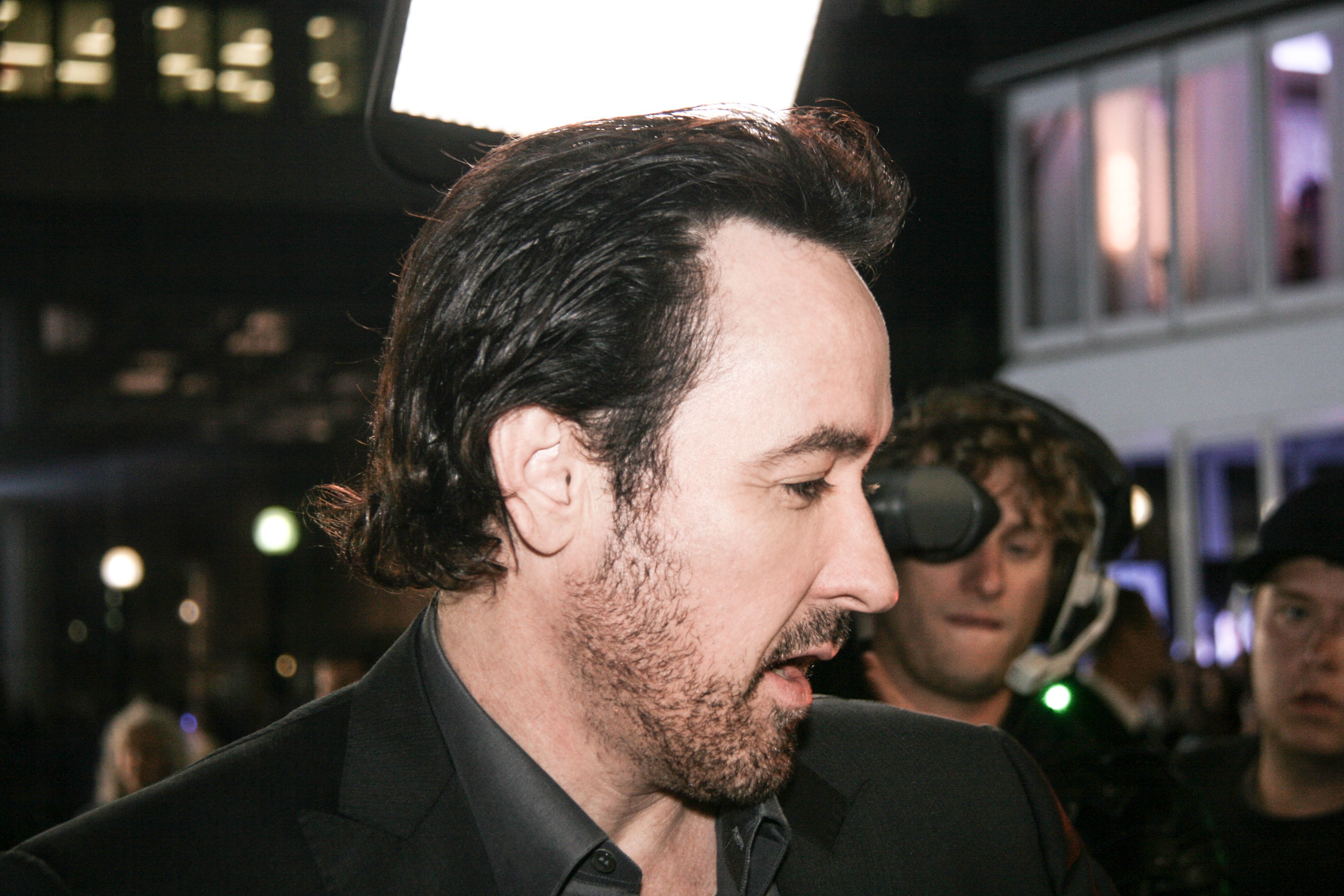The photograph is a close-up side profile of John Cusack, who is looking to the right. He is dressed in a black suit jacket over a black undershirt, complemented by his short brushed-back brown hair and a light beard and mustache. Behind him, the background is a bit dark and out of focus, but distinctly notable are two men, presumably part of a film crew. One man is operating a camera, with a large over-the-ear headset that has a microphone in front of his mouth, while the other man, wearing a black baseball cap, looks on. A large, square-shaped light is situated above Cusack’s head, indicating an on-set environment. To the right in the background, there is a somewhat blurred view of buildings, with light shining through windows, suggesting an outdoor, daytime setting. Various colors including black, white, shades of gray, tan, green, pink, and purple are present in the image, although the specifics are less clear due to the blurriness.